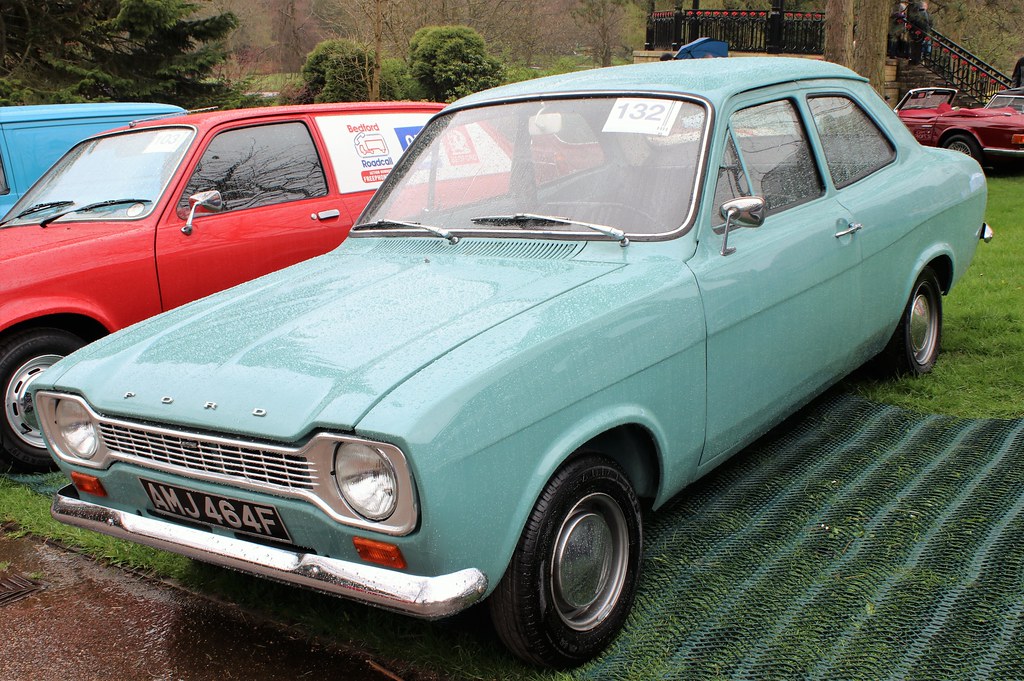In this detailed image, we see a collection of vintage cars parked on a grassy surface, evoking a nostalgic scene possibly set in the UK, given the wide, long European-style license plates. Dominating the foreground is a baby blue, antique Ford, distinguished by its silver Ford letters on the hood and the license plate reading AMJ464F. This light blue car, likely from the 1950s or 60s, is angled with the driver’s side on the right, and is positioned on top of a green mesh mat beside a cement curb, possibly for practical reasons to protect the grass.

Next to the vintage Ford is a red, miniature van, also looking slightly aged but not as much as the blue Ford. Near the red van is an aqua van, adding more hues to the antique ensemble. Further in the background, under a veranda leading up to a building, sits a red convertible, its top down despite the apparent rainfall. The scene suggests a classic car show, complete with a staircase leading up to a canopy and netted matting visible in the bottom right-hand corner of the image, hinting at a well-organized display setting.